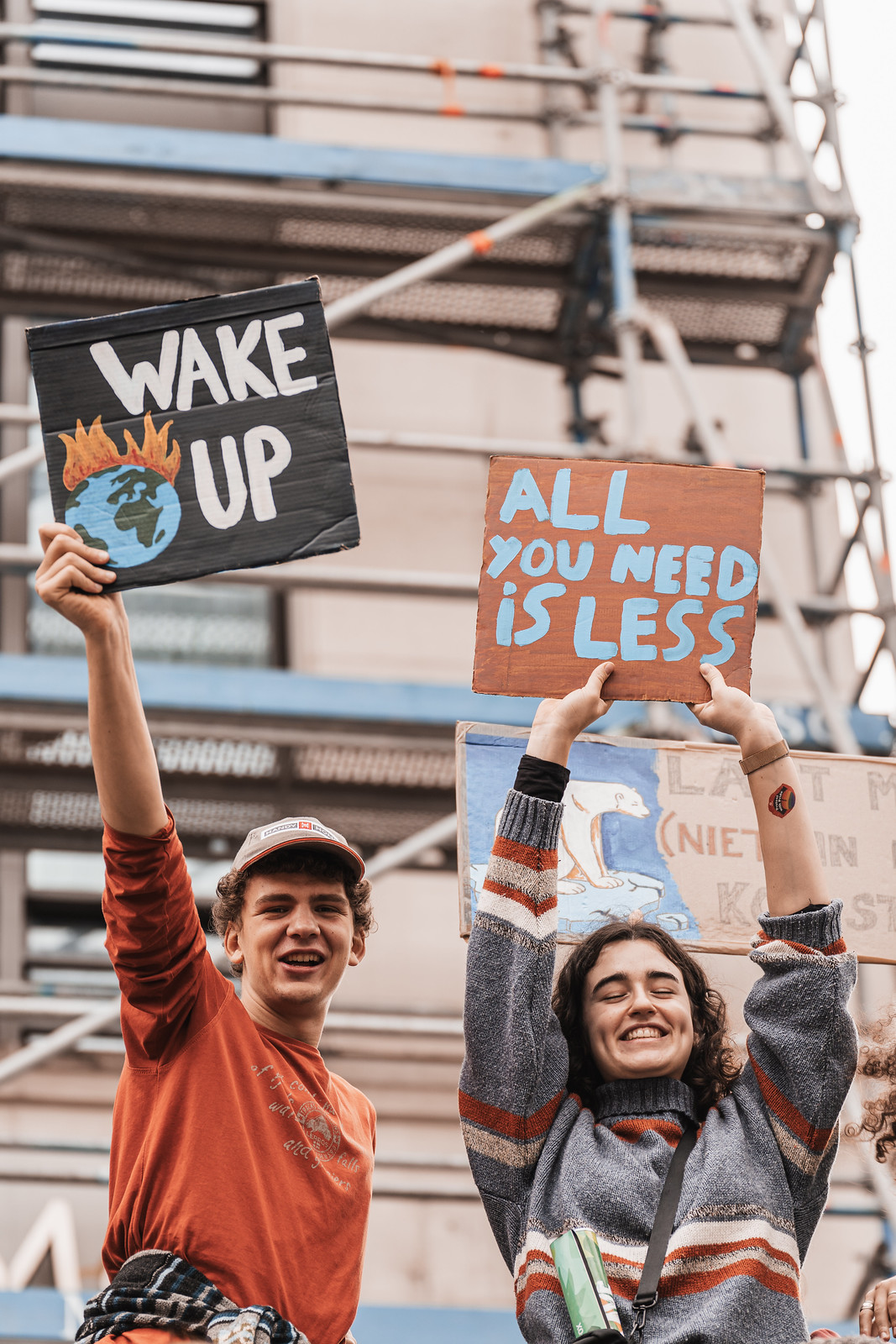In this daytime photograph, two young individuals, likely in their late teens or early twenties, stand waist-up in front of a tall building undergoing construction. The person on the left is a man wearing an orange long-sleeve t-shirt, a light gray hat, and a checkered shirt tied around his waist. He holds a black sign with white text that reads "WAKE UP," featuring an image of the Earth engulfed in flames. The woman beside him is dressed in a woolen sweater with red, white, and blue stripes. Her left arm, which displays a tattoo and a watch, is partly exposed. She holds a brown sign with blue text that says "ALL YOU NEED IS LESS." Both are smiling, with the woman displaying dimples and closed eyes. In the background, construction railings and a glimpse of the sky are visible, hinting at their presence at a protest, possibly related to climate change or pollution, although the signs behind them are unreadable. The color palette of the image includes black, white, gray, orange, brown, blue, green, red, and shades of off-white.